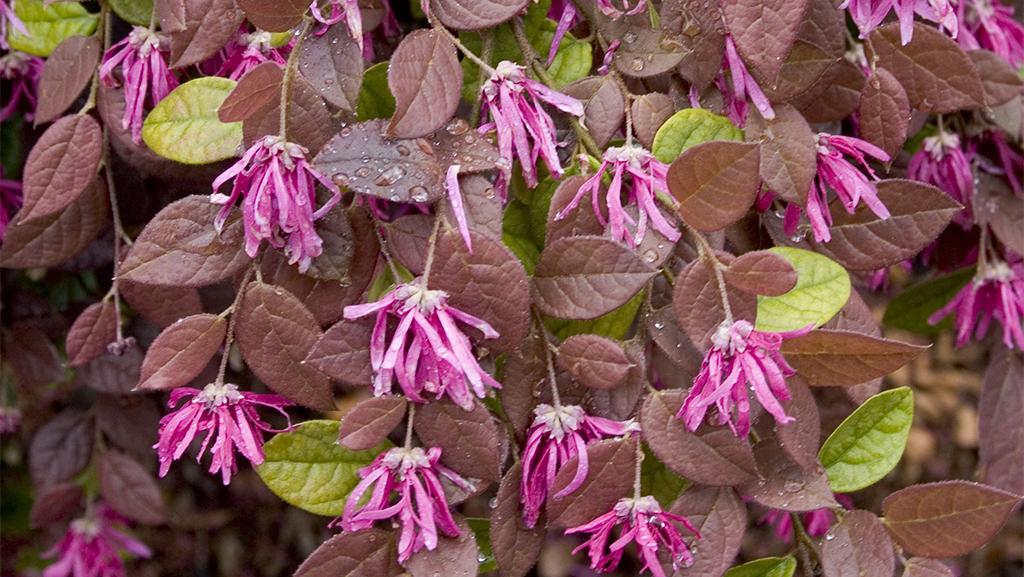The image is a detailed outdoor photograph taken during the daytime, capturing a flowering vine or bush in full view. The composition is rectangular, approximately five inches wide and three inches high, showcasing an intricate close-up of the plant. Dominating the foreground are delicate, drooping pink flowers with long, narrow petals and light pink undertones. These flowers are connected by thin stems or vines, from which elliptical-shaped leaves emerge. The leaves display a variety of colors; while many are a reddish-brown, several light green leaves can also be seen intertwined. Water droplets are delicately scattered across both the leaves and petals, adding a fresh, dewy appearance. In the background, more flowers and leaves are visible, with some appearing out of focus, enhancing the depth and lushness of the scene. The pink flowers, possibly razzleberries or razzleberry fringe flowers, are interspersed throughout, creating a vivid contrast with the reddish-brown and green leaves.